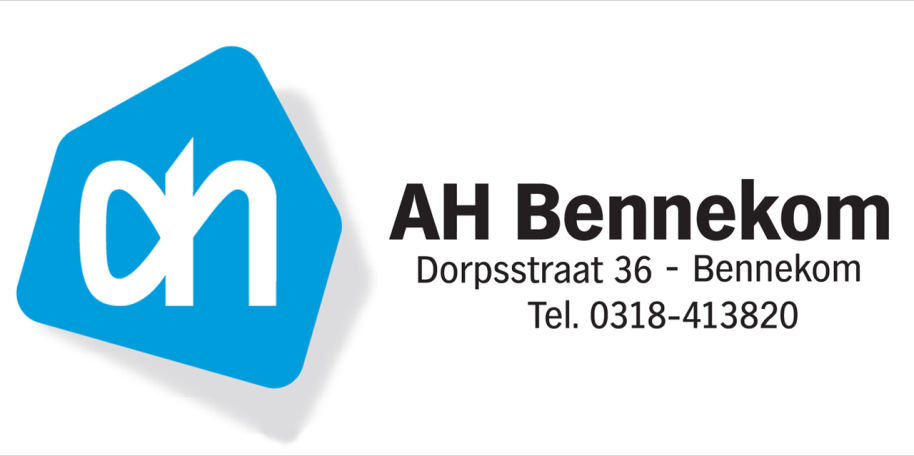The image likely depicts a business card or advertisement centered within two thin gray horizontal lines, one at the top and one at the bottom, on a white background. On the left-hand side, there is a large blue pentagonal logo resembling a house with a rounded top and bottom corners, tilted slightly to the right. Inside the logo, there are white letters "H" connected to an "N". To the right of the logo, in large, bold black text, the company name "A H Benekom" is written. Below this, in smaller black text, are the details: "Dorpstraat 36 - Benekom" and "TEL. 0318-413820", all center-aligned. The text suggests the address and phone number are likely in a Dutch context.